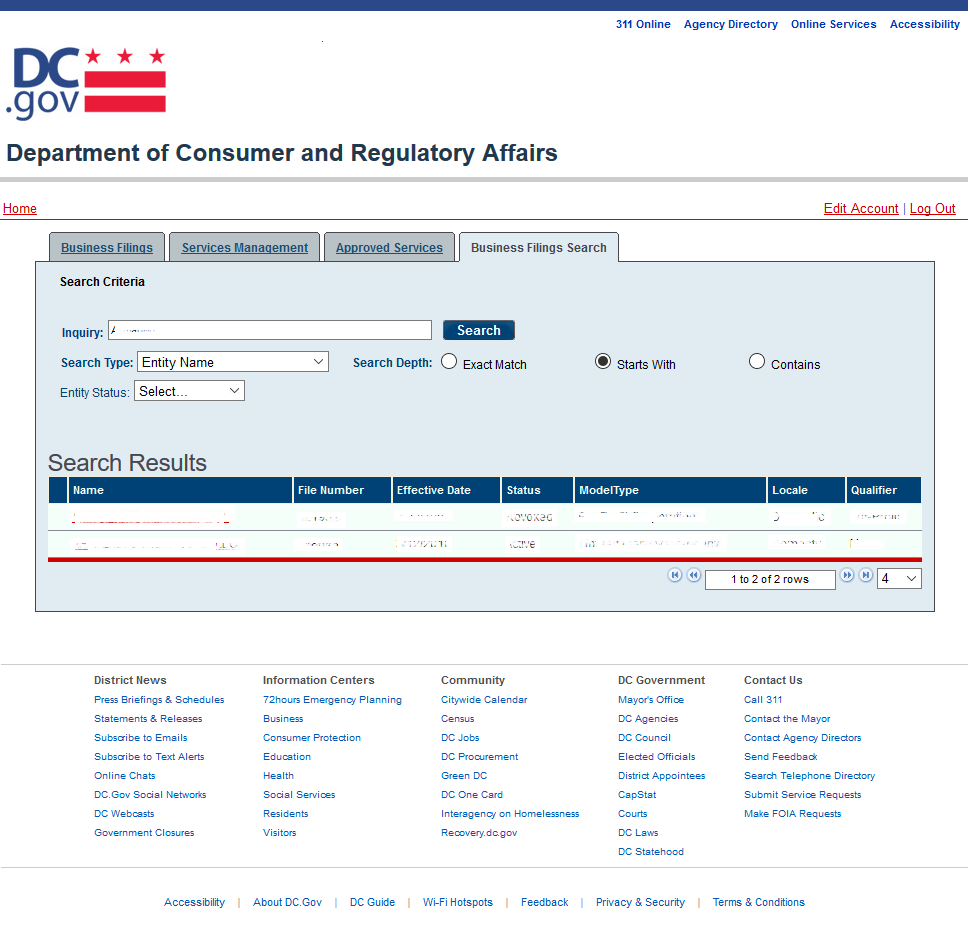The image features a screenshot of the DC.gov web page, specifically from the Department of Consumer and Regulatory Affairs. Prominently displayed at the top are links to various resources including Copyrights, 311 Online, Agency Directory, Online Services, and Accessibility. The navigation bar includes options for Home, Edit Accounts, Logout, and additional links.

Below the navigation, the page is focused on business-related services with sections like Business Filings, Services Management, Approved Services, and Business Filing Search. The search panel provides multiple search criteria options including Search Type, Entity Name, and Entity Status with dropdown menus for specifying the search depth. Notably, the "Exact Match" and "Contains" options are visible, with "Stats Suite" being selected for the search depth.

On the right side, additional informational links are displayed under District News, Information Centers, Community, D.C. Government, Contact Us, Privacy and Security, Wi-Fi Hotspots, D.C. Guide, and details about the website's accessibility features.